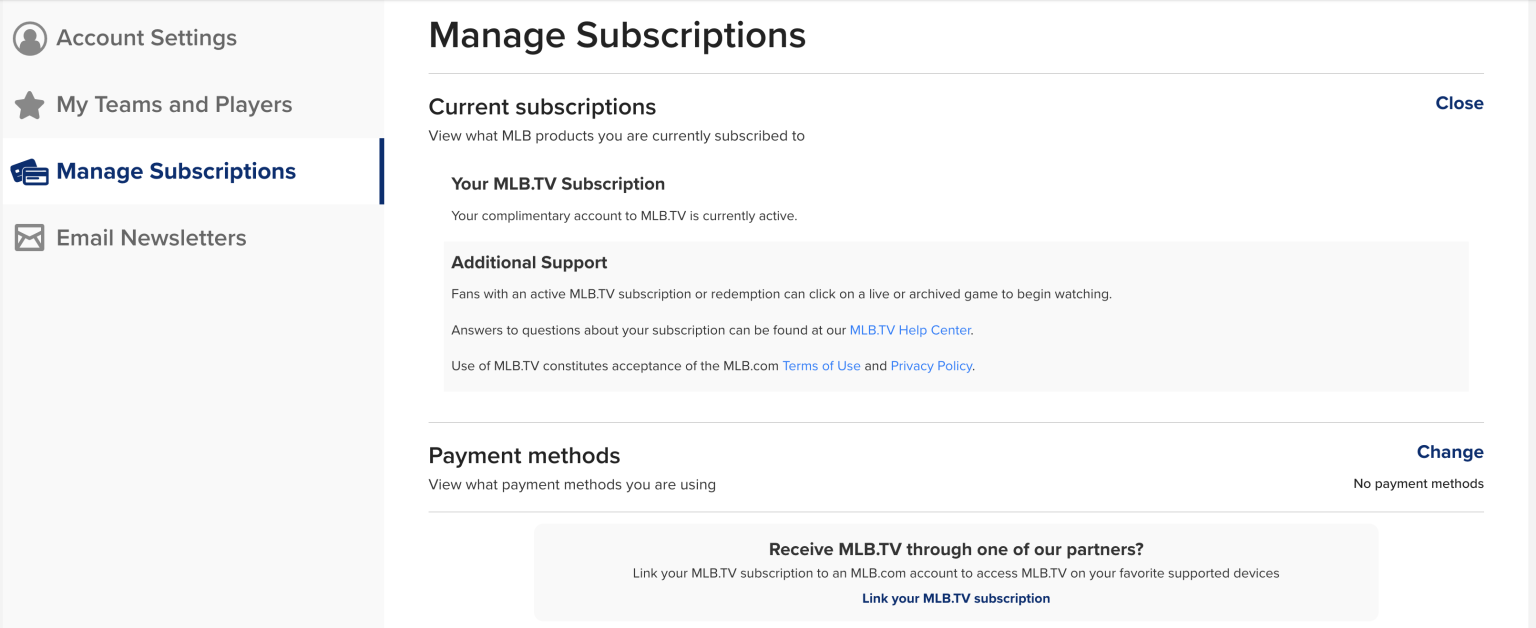The image is a screenshot of a settings page on a website, which is divided into several categories listed on the left side. The first category is "Account Settings," followed by "My Teams and Players," "Managed Subscriptions," and "Email Newsletters."

The viewer is currently in the "Managed Subscriptions" tab. At the top of this section, the header reads "Managed Subscriptions." Directly beneath this, there is a subsection titled "Current Subscriptions," which indicates that the user is subscribed to MLB products. Specifically, it mentions that the user has an active complimentary account to MLB.tv.

Below this, there are additional headings: "Additional Support" and "Payment Methods." Under "Payment Methods," it states that there are no payment methods currently associated with the account. To the right of this information, there is an option labeled "Change" for updating payment methods.